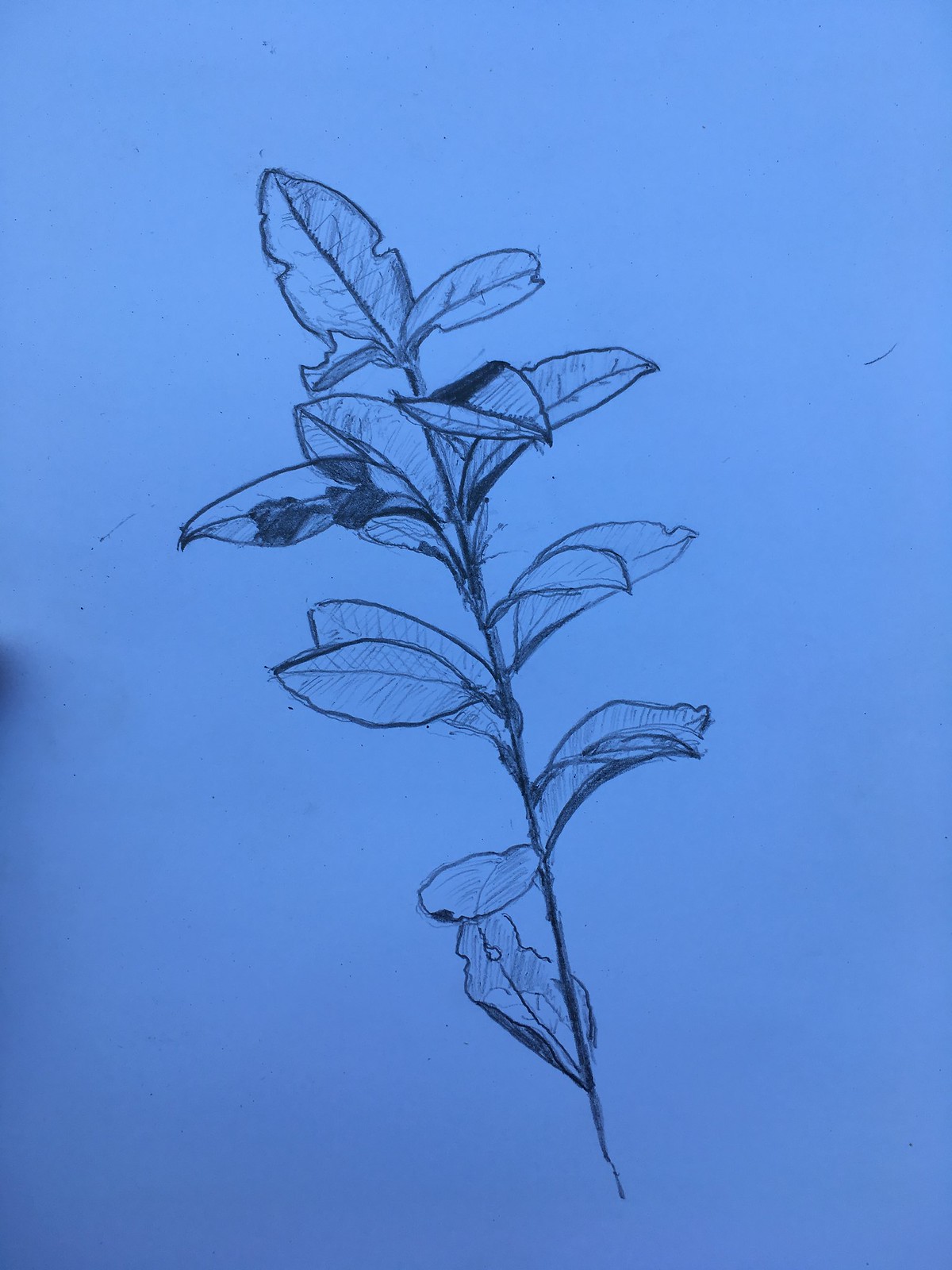The image showcases a meticulously detailed pencil sketch set against a light blue background. The sketch features a slender stem or thin branch adorned with a series of almond-shaped leaves. Starting from the base, there is a solitary leaf extending to the left. Ascending from there, the branch exhibits approximately 10 leaves in total.

One of the uppermost leaves stands almost straight up, slightly bent to the left, exhibiting signs of being chewed by insects or possibly suffering from disease. A similarly damaged leaf appears just below it, also showing chewed edges. As we move further down the branch, the leaves become progressively fuller and healthier in appearance. The artist’s attention to detail in capturing the various textures and conditions of the leaves adds depth and realism to this botanical study.